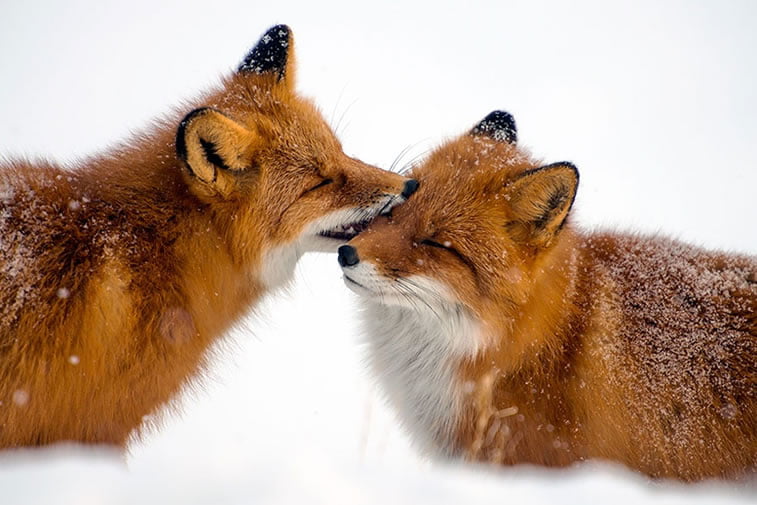This engaging photograph captures a heartwarming scene of two red foxes playfully interacting in a snowy landscape. The image is horizontal and rectangular, with a white background that emphasizes the cold, wintry setting. At the center of the frame, the fox on the left gently nibbles or nuzzles the face of the fox on the right, evoking the tender feel of an Eskimo kiss. Both foxes have reddish-brown fur, thick and fluffy, with distinctive black edges around their ears and white fur extending from the bottoms of their noses down across their necks. Their eyes are closed, adding to the affectionate atmosphere. Light snowflakes are visible on their backs and ears, adding a delicate touch to this charming moment.